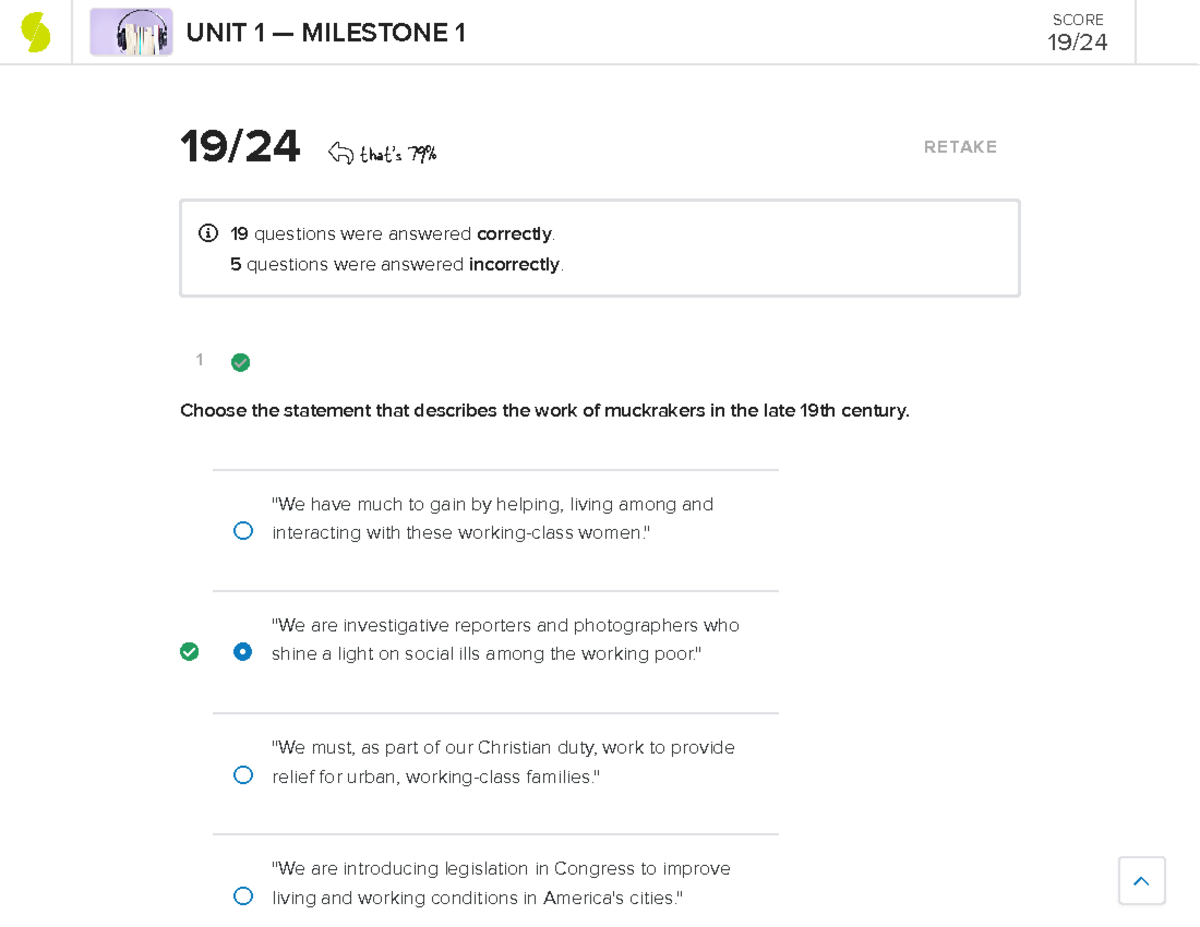On an all-white background, the image features various elements arranged systematically. In the top left corner, there are two yellow half-circles. The left half-circle is slightly above the right one and is tilted slightly to the right. Below these shapes, a line extends horizontally all the way to the right, accompanied by a thin gray line parallel to it.

To the right of the lines, there is an image of headphones set against a blue background. Adjacent to the headphones image, in bold black capital letters, it reads "UNIT 1 - MILESTONE 1." On the far right side of the image, the word "SCORE" is displayed, and directly underneath it, the score "19/24" is written.

Beneath the "UNIT 1" text and the horizontal line, the score "19/24" is displayed again in bold, with an arrow pointing to the left towards it. Next to this score, in smaller black lettering, it states "That's 79%". On the right side of this section, there's a button labeled "RETAKE."

Further down, there is a rectangle with a gray border enclosing a white circle with a black border and an exclamation point inside it. It reads, "19 questions were answered correctly." Below this, it notes, "5 questions were answered incorrectly."

Moving downward on the left side of the image, the number "1" is displayed alongside a green circle with a white checkmark inside it. This section includes the text, "Choose the statement that describes the work of muckrakers in the 19th century." A thin gray line separates the question from the answers below.

Below this line, there are multiple-choice options indicated by circles and lines. The first option has a white circle with a blue border, followed by two horizontal lines—a characteristic of an option in this format. The second option features a blue circle with a white center to the left of a green circle with a white checkmark, indicating the correct answer. The subsequent two options have the same white circle with a blue border and two lines beside them, signifying additional choices.